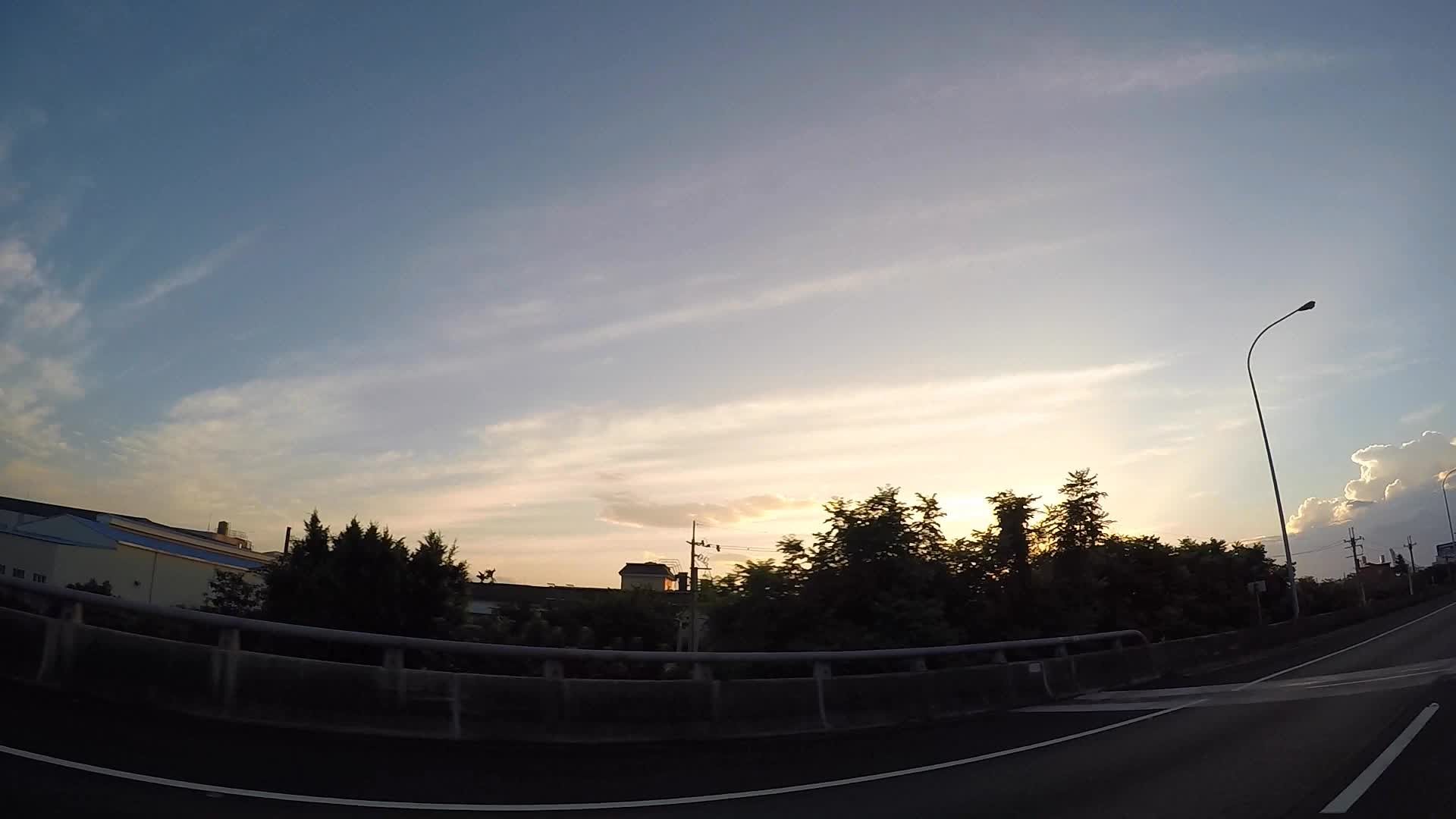A serene suburban scene bathed in the warm hues of a setting sun unfolds in this photo. The sun, on the verge of disappearing below the horizon, casts its final golden rays through scattered clouds, creating a dramatic interplay of light and shadow in the sky. Below, a quiet residential street stretches out, bordered by a tree line that partially obscures a few buildings, their outlines softened by the foliage. A street lamp stands sentinel beside a road that's lined with telephone wires and a railing that hints at a nearby bridge. The vantage point from the street offers a grounded perspective, directing our gaze upwards to the vivid blue sky being gradually consumed by the encroaching twilight. The entire scene evokes a tranquil moment of transition as day gives way to night.